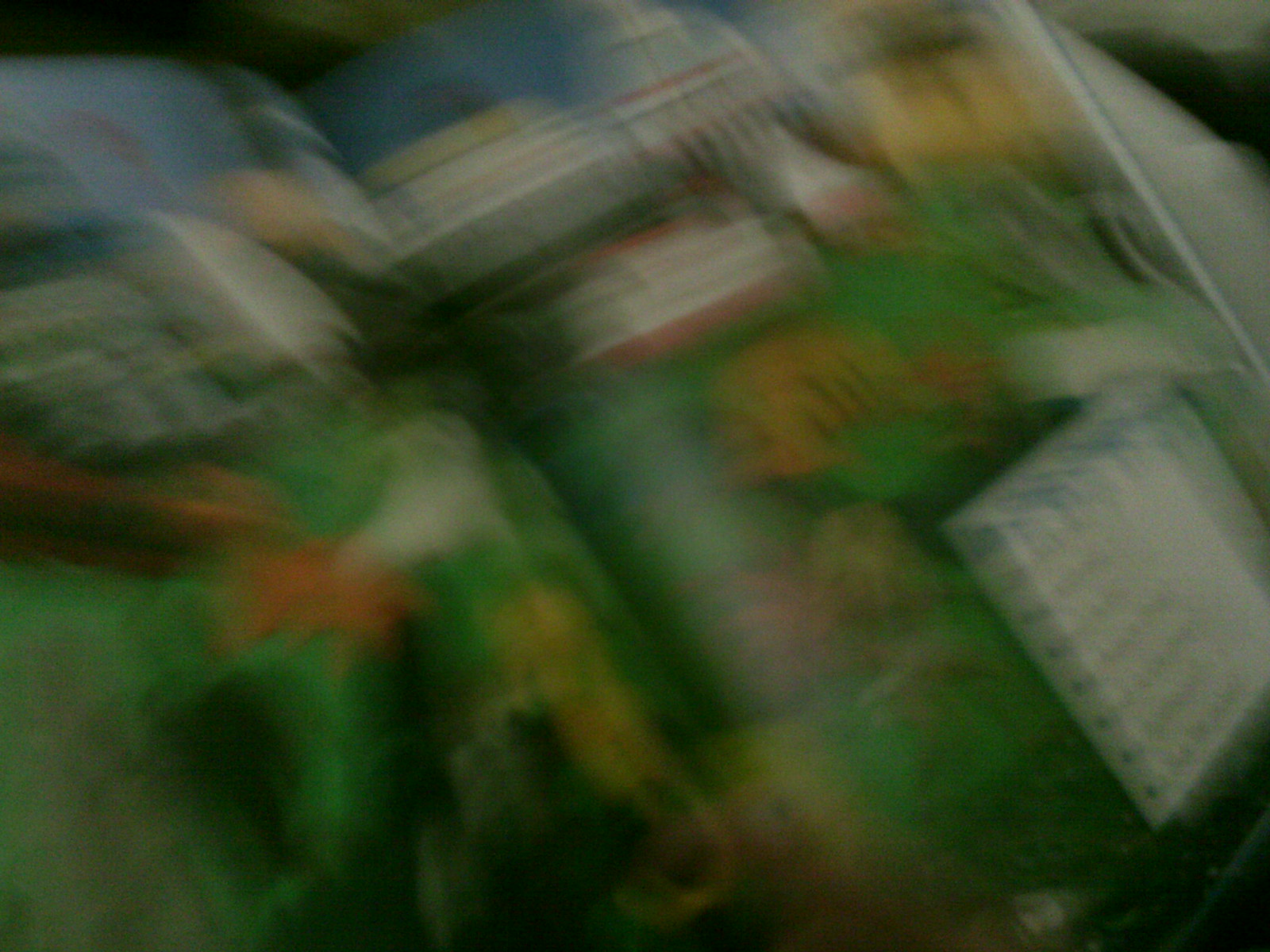A very blurry image shows an open book, with two colorful pages on display. The bottom right corner features a white square containing lines of text, possibly serving as a key or legend. The image predominantly shows a green hue, interspersed with orange patches that could resemble flowers. Near the top, blurred shapes suggest a line of boats against a blue background, likely representing the sky. One boat, in particular, has a red bottom and a white interior, though the details are obscured by the blurriness. The overall composition seems to depict a scene abundant with plant-like elements.